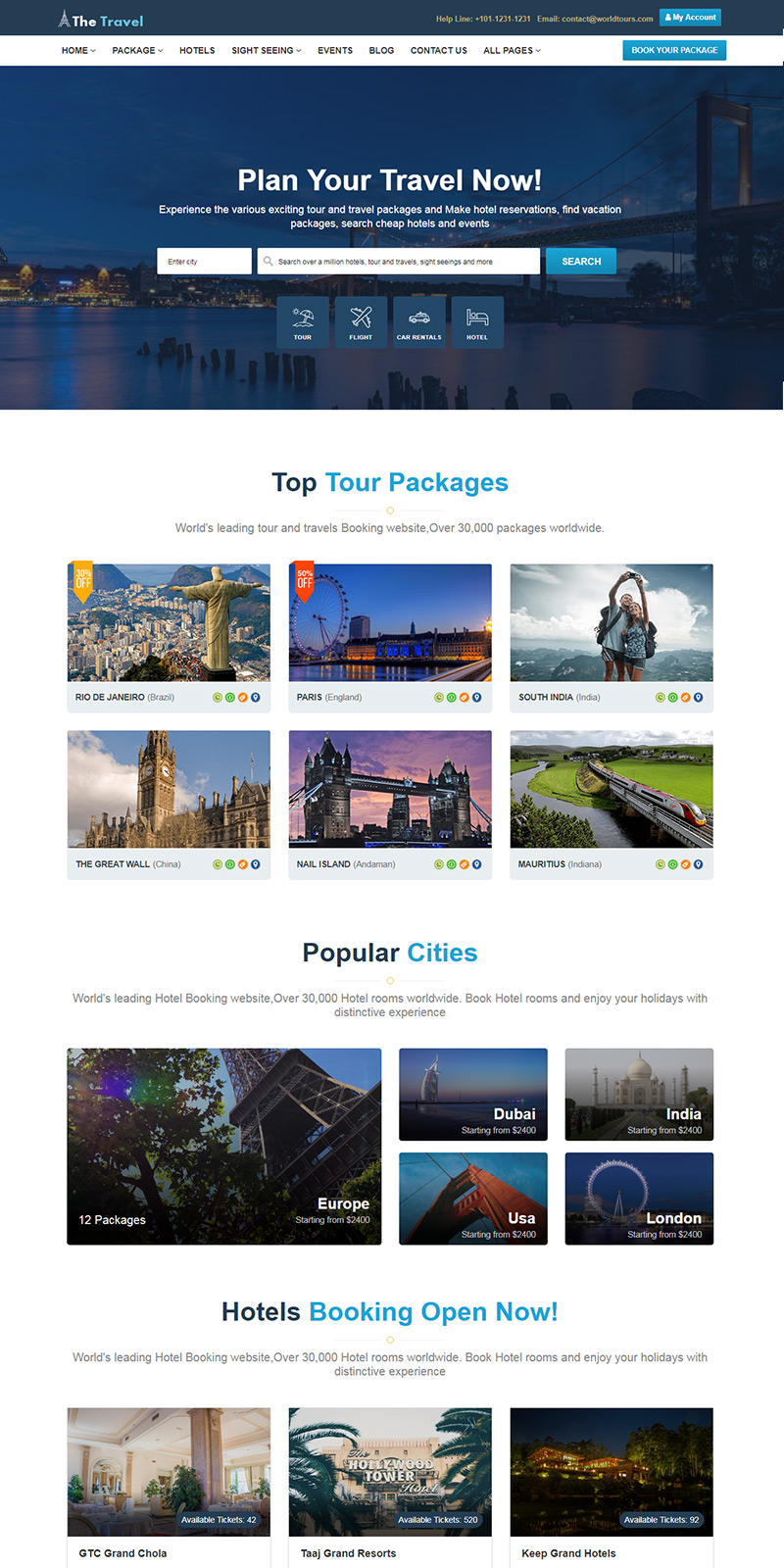**Website Screenshot Overview**

This screenshot captures the interface of a travel-themed website, featuring a structured layout with various interactive elements and vibrant imagery.

- **Header Section:**
  - A navy blue navigation bar spans the top of the page, adorned with white and light blue text. The text reads "The Travel," although the latter part of this is somewhat blurry. An icon resembling the Eiffel Tower is situated nearby, enhancing the travel motif.

- **Main Interface:**
  - **Sidebar on the Left:**
    - Contains multiple submenu items displayed in a navy blue format.
  - **Content Area:**
    - A light blue and white call-to-action box prominently features the message "Plan your travel now," accompanied by brief descriptive text.
    - Below this box, there are two gray and white search boxes, each equipped with a magnifying glass icon for search functionalities.
    - Another blue and white box appears, alongside four blue squares each depicting distinct icons: a beach umbrella, an airplane, a car, and what is likely a bed.

- **Featured Sections:**
  - **Top Tour Packages:**
    - This section's header is highlighted in blue, with a short description in gray text. It showcases a lineup of captivating images:
      - The iconic Christ the Redeemer statue in Brazil, marked with a gold banner.
      - A ferris wheel adjacent to a body of water, flanked by an orange banner.
      - Two people hiking and taking a selfie, illustrating adventure and leisure.
    - Beneath these images are various colorful icons in green, orange, and blue.

  - **Popular Cities:**
    - Highlighted by a blue header, this section includes a short descriptive text.
    - Images featured:
      - A partially visible Eiffel Tower labeled "Europe."
      - An architectural landmark in Dubai.
      - A partial view of the Golden Gate Bridge in the U.S.
      - A temple in India.
      - A ferris wheel in London.

  - **Hotels Booking Open Now:**
    - Clearly demarcated by a blue header and accompanied by brief text.
    - Displayed images include:
      - A stylish hotel lobby.
      - Palm trees flanking a building.
      - A building illuminated at night.

This detailed visual tour through the website's interface aims to convey the thrill and variety of travel options available, enticing users to explore and plan their journeys.